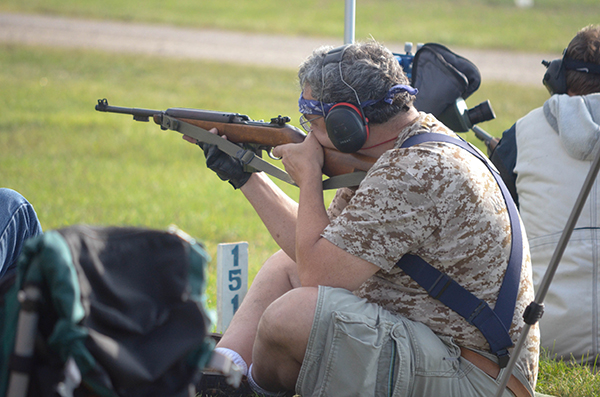The photograph captures a competitive shooting event featuring several participants seated closely together on a grassy field. The central figure, identified by the participant number 151 displayed on a wooden placard in front of him, is a fair-skinned man intently aiming a brown rifle. He is equipped with protective ear muffs and glasses, while a blue bandana, presumably to keep sweat out of his eyes, is wrapped around his forehead. He wears a desert-style urban camo t-shirt in tans and browns, paired with khaki cargo shorts and a brown leather belt. Shooting gloves cover his right hand, ensuring a steady grip on the rifle. Other participants can be seen sitting on either side of him, indicating the camaraderie and competitive spirit of the event. The scene is set against a background of lush grass and a dirt trail or roadway running through the upper part of the image, adding context to the outdoor setting.